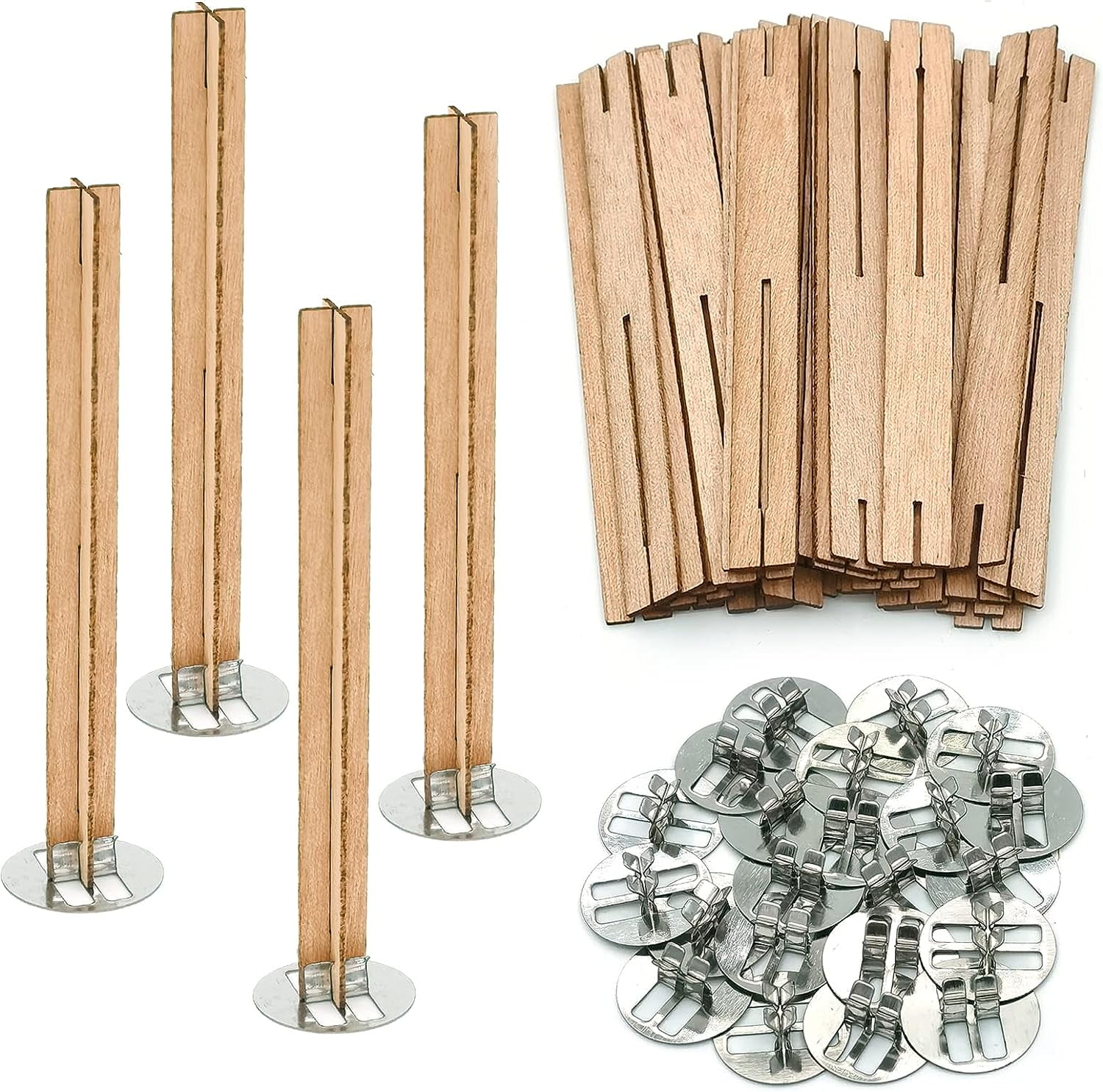The image comprises three sections arranged on a white background, with one section on the left and two on the right. The top right section features four brown wooden sticks, each with slits at their top and bottom ends, and holes along their bodies. The slits are shorter at the top and longer at the bottom. These wooden sticks are paired with shiny, silver metallic bases that are round and have extensions on their surfaces. In the bottom right section, multiple silver bases are displayed, showcasing their circular shapes and metallic sheen. The left section of the image presents an assembled structure where the wooden sticks and metallic bases are combined. This structure stands straight and self-sufficiently, with a metallic base at the bottom and wooden sticks attached to it, suggesting it could potentially function as a tool, book holder, napkin holder, or possibly table legs.